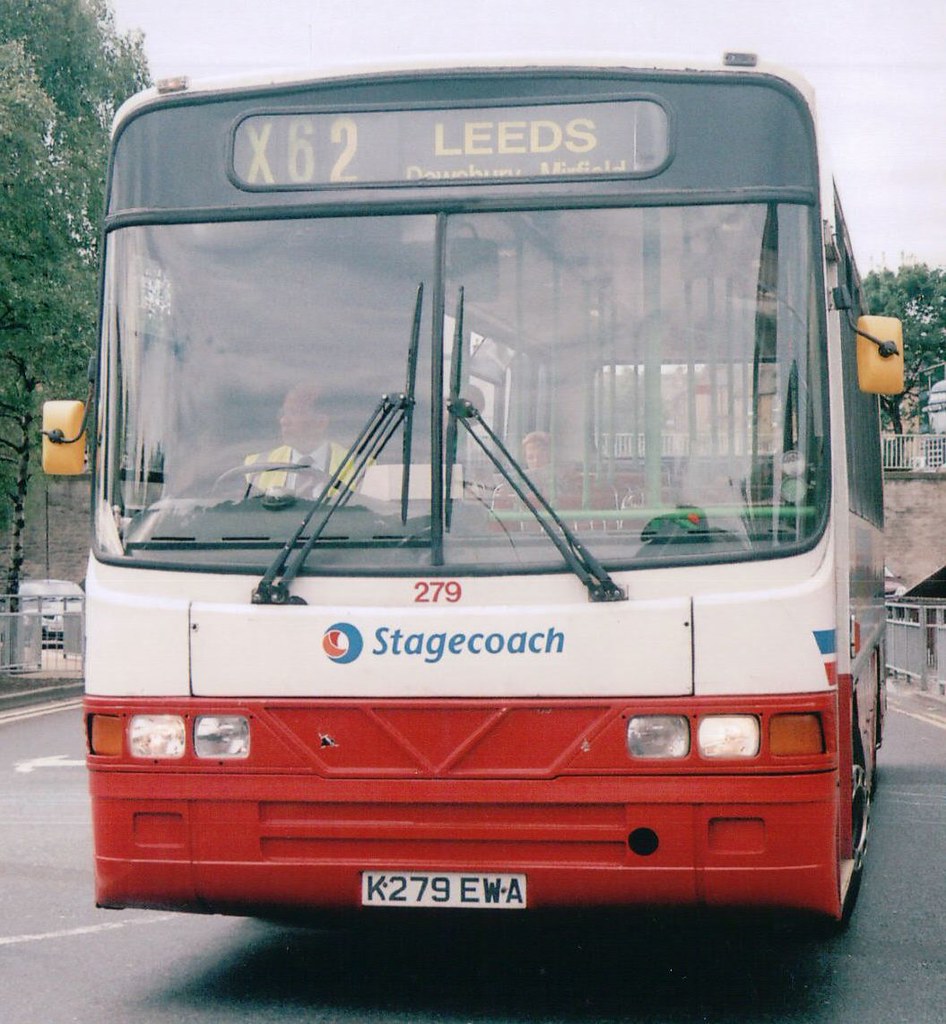This photograph captures the front view of a Stagecoach bus with a striking white body and a red base. The bus prominently displays the identifier "279" across its center, alongside the Stagecoach logo to the left. The LED banner at the top of the bus reads "X62 Leeds Devonbury Midfield," although part of it appears to be partially rolled down. The license plate reads "K279 EWA." The bus driver, situated on the right side of the bus due to the left-hand driving norm in England, is visible through the windshield, wearing a white shirt and a yellow high-visibility vest. 

The scene is set outdoors on an overcast day, evidenced by the hazy light and the overcast sky visible at the top and right corner of the image. Green trees frame the left side, suggesting it was likely taken in spring or summer. Below and to the left of the bus, a metal fence and some pavement are noticeable, and beyond the bus, there appears to be a road or parking area with cars. The bus is equipped with yellow side mirrors, and the light reflection on the windshield adds a dynamic touch to the overall composition.